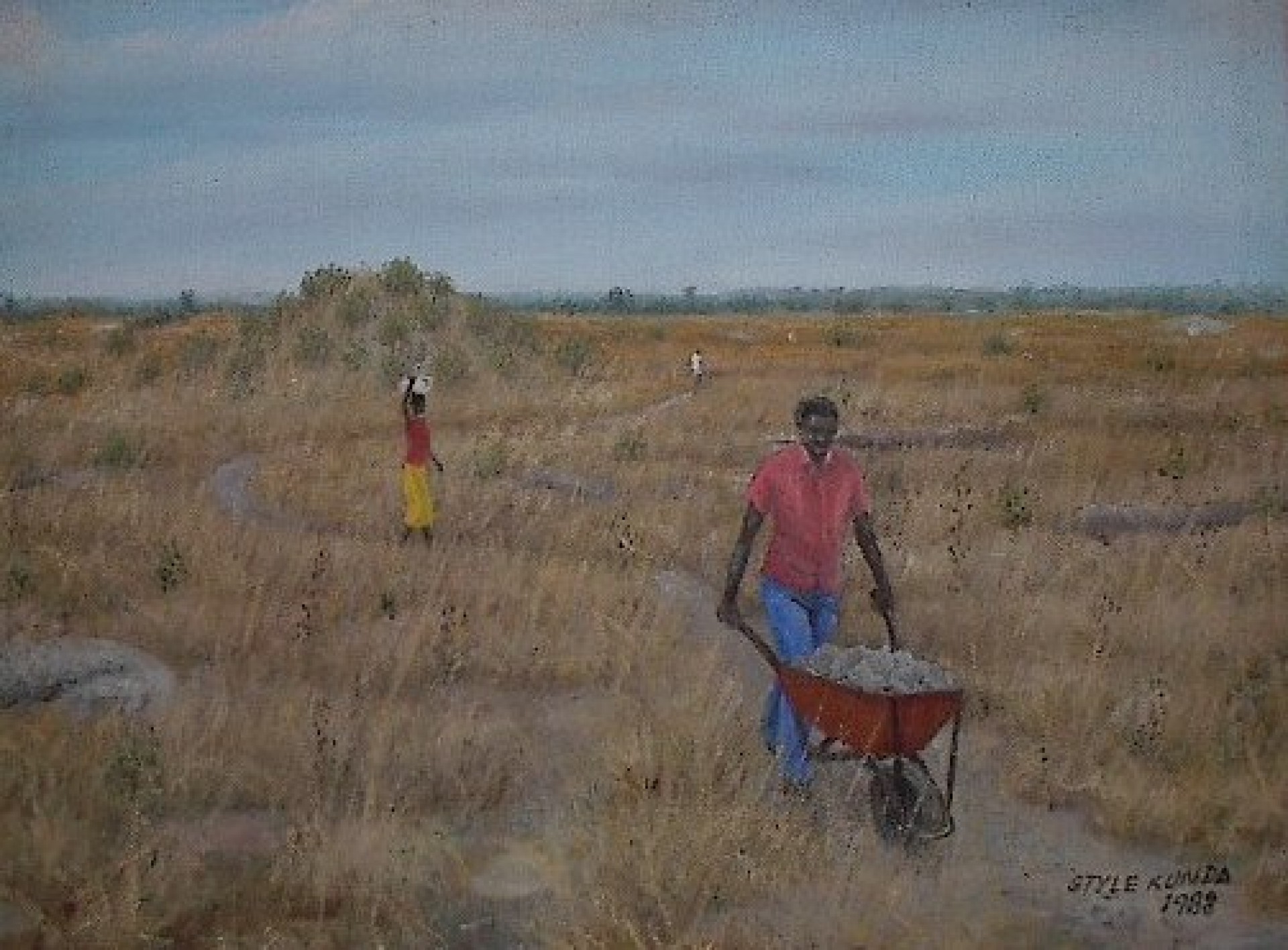This detailed illustration, reminiscent of a painting, depicts a scenic evening in a wide-open field characterized by earthy tones of green, brown, and tan. The foreground features a black man wearing a red shirt and blue jeans, pushing an orange wheelbarrow loaded with gray rocks along a winding gray path. Further back, a figure in a red shirt and yellow pants balances a white object on their head with their right hand for support. The winding path leads past patches of grass, dirt, and tan weeds, eventually reaching a small hill with sparse drab green bushes. In the hazy, cloud-filled blue sky, the painter's signature "Tyle Kunda 1988" is visible in the bottom right corner. A person in a white shirt can be seen far in the background, adding depth to the artwork.